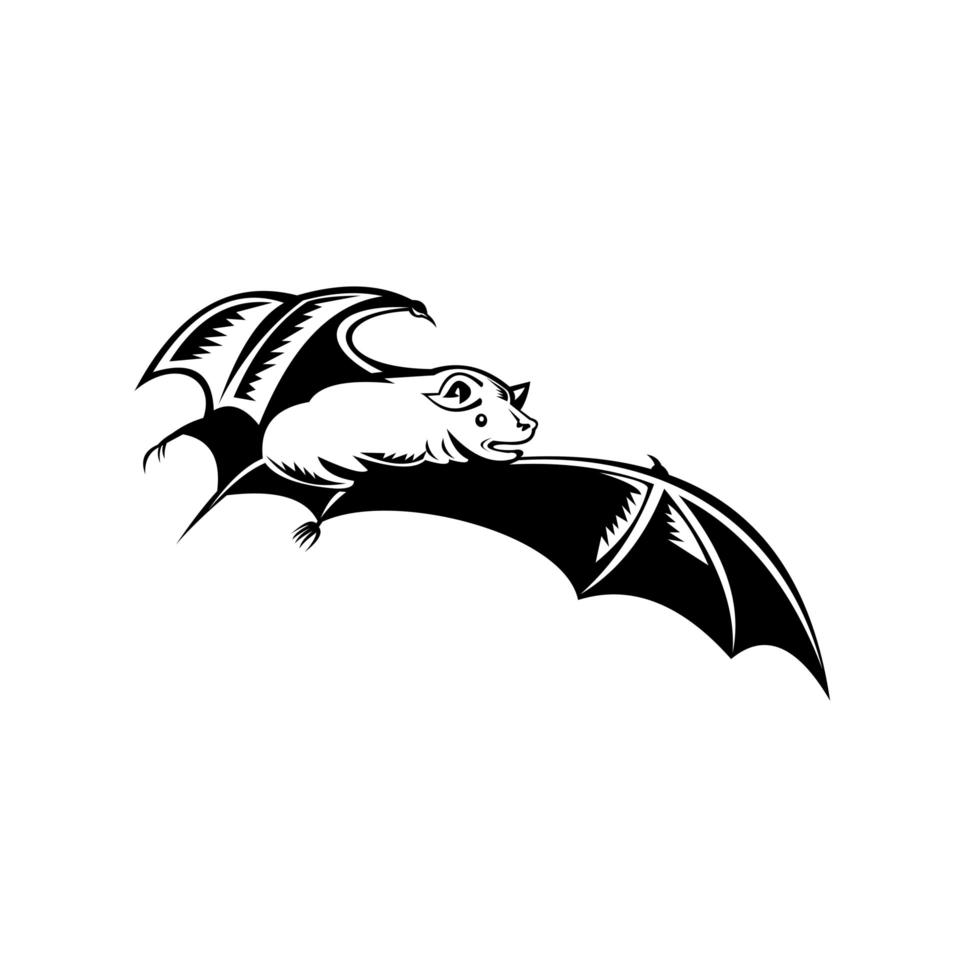This is a black and white PNG-style vector art of a bat in flight, facing to the right. The image, which could be used as a logo or clip art, is set against a plain white background with no additional elements. The bat's wings are bold and black, featuring a traditional semicircular design with perforated edges and white stripes or separations between them. The nearer wing appears slightly folded over, enhancing the sense of motion. The bat's face, which has a small smile, pointy ears, and an open mouth as if emitting a sound, is oriented towards the right. Additionally, the bat has a thin, rat-like tail and a sharp thumb at the end of each wing.